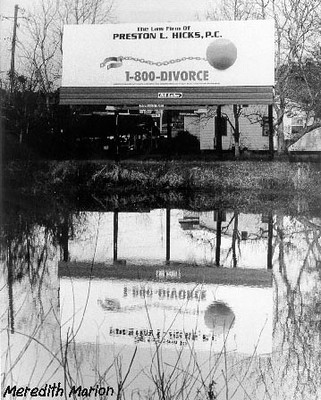This detailed black-and-white photograph captures a rural outdoor setting, featuring a large billboard prominently in the top third of the vertical frame. The billboard advertises the law firm of Preston L. Hicks, P.C., displaying a striking image of a broken ball and chain and the phone number "1-800-DIVORCE." The billboard stands before a reflective canal that beautifully mirrors its image along with surrounding elements. In the background, the scene includes a white clapboard house and several leafless trees, adding to the stark, wintry atmosphere. The lower left-hand corner credits the photographer, Meredith Marion, emphasizing the professional quality of the image.